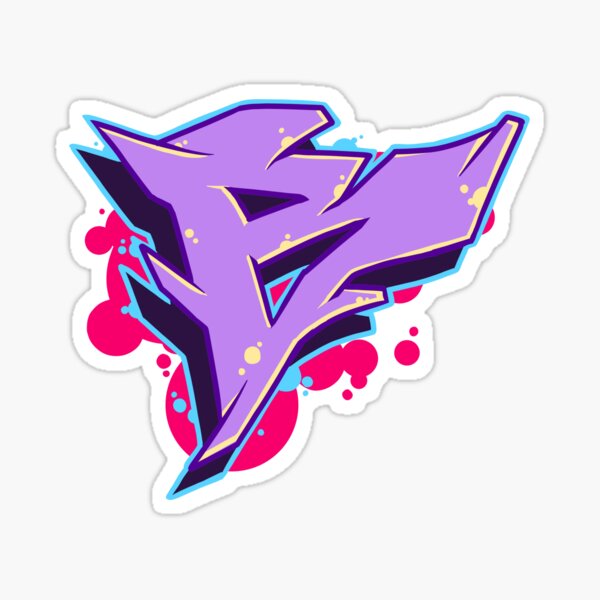The image is a large square with a light gray or off-white background. In the center, there is a prominently displayed, artistic capital "B." This "B" is primarily purple, with decorative gold circles scattered throughout its form. It features unique cutout sections shaped like triangles, with the inner edges of these cutouts highlighted in dark blue and accented with gold. 

Surrounding the "B" is an intricate border and background. The immediate outline around the "B" is gray, shaded with white, contributing to a three-dimensional effect. Additionally, there are distinct red and reddish-pink round shapes positioned to the left and bottom side of the "B," enhancing the graffiti-like aesthetic. There are no other texts or markings in the picture, making the "B" the central focus of this computer-generated graffiti artwork.